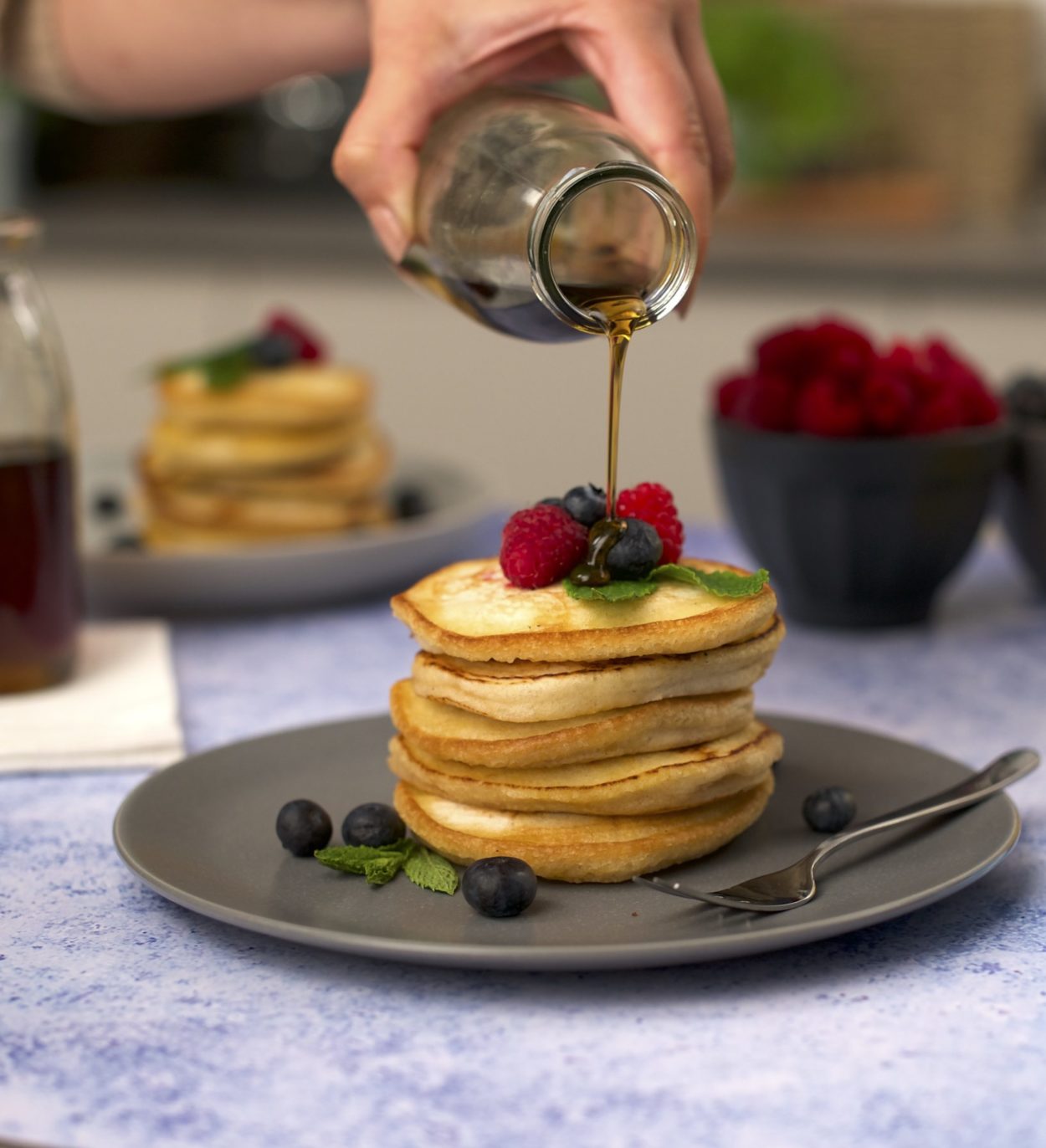In this detailed, horizontally-oriented photograph, we see an indoor setting centered around a gray plate holding a stack of six thick pancakes. The pancakes are topped with fresh blueberries and raspberries, with a few blueberries scattered around the base on the plate. A woman's hand, just off the top of the image frame, is pouring syrup from a clear, milk jar-style container onto the pancakes. A silver fork rests on the plate in the foreground. The setup rests on a blue and white mottled tablecloth. In the background, out of focus, are additional breakfast items: another stack of pancakes also adorned with berries to the left, accompanied by another jar of syrup, and two dark gray bowls to the right, filled with raspberries and partially-visible blueberries. The entire scene exudes a cozy, inviting breakfast atmosphere.